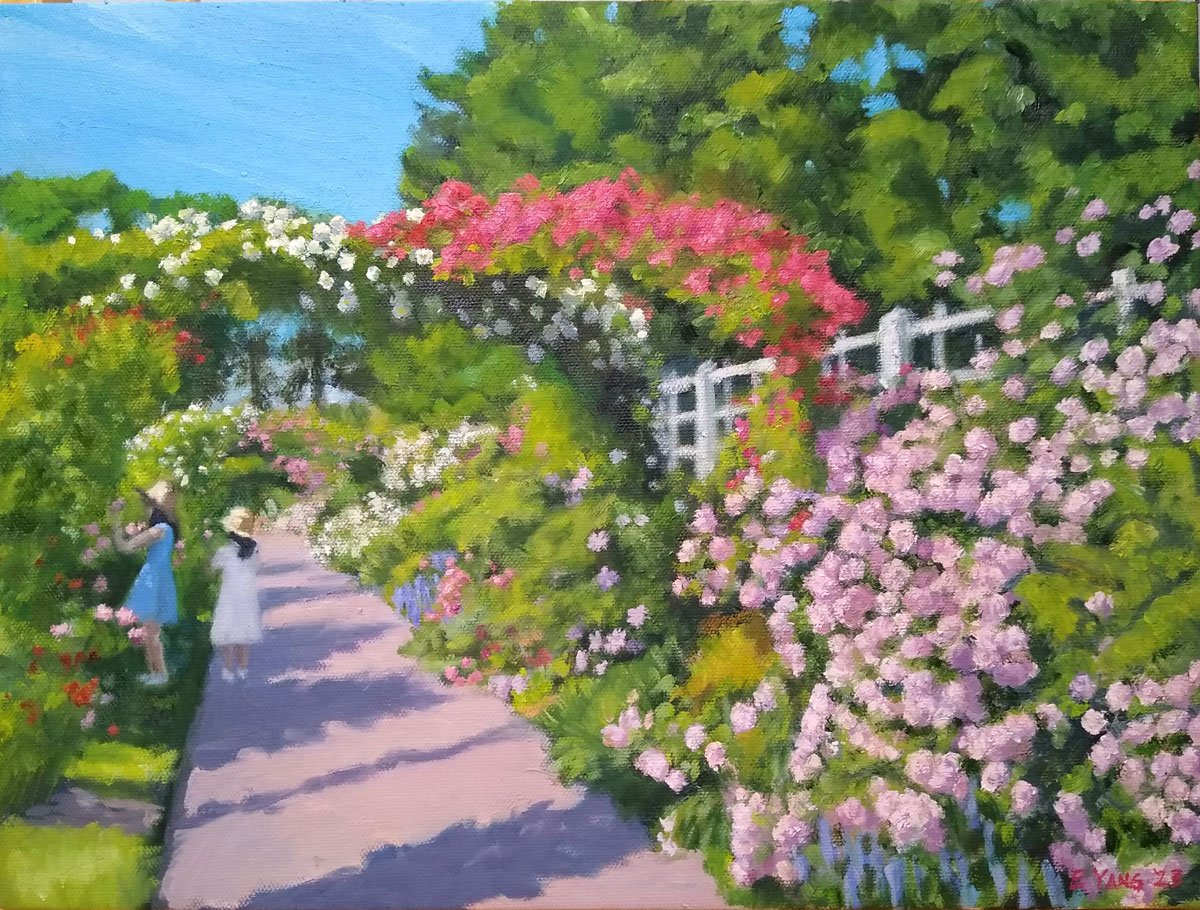This watercolor painting on canvas depicts a serene flower garden in summer, where two young girls stand on a paved path that winds through several arches of flowers. The scene is bathed in subtle, subdued colors, emphasizing the delicate beauty of the garden. The path, flanked by blooming flowers and shrubs in shades of pink, lavender, and white, leads to the background where fully grown trees and a cloudless blue sky provide a tranquil backdrop. The two girls, both wearing large hats and white shoes, are absorbed in the beauty around them: one is dressed in a blue dress and the other in a white dress. Both appear to be engrossed by the flowers they are closely observing. A small white fence is intermixed with the floral display, and shadows cast by unseen trees add depth to the composition. The overall effect is one of gentle charm and natural elegance, suitable for an art gallery.